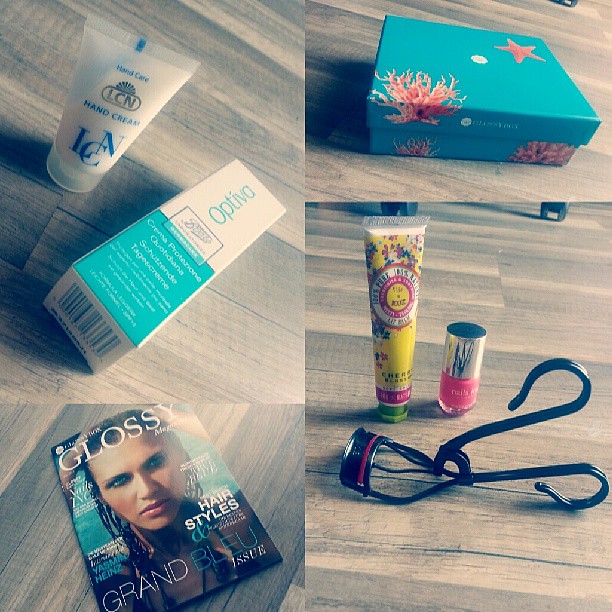The image is a collage divided into four squares, each featuring various items on a wooden floor. In the top left square, there is a white bottle of hand cream labeled "LCN" with blue lettering, and next to it is a white and teal box reading "Optiva." The bottom left square showcases a magazine titled "Glossy," with a woman's face on the cover and the words "Grand Bleu" at the bottom. In the top right square, there is a turquoise-blue shoebox adorned with images of a pink coral and a pink starfish. Finally, the bottom right square displays three items: a yellow bottle with a green cap, a small pink nail polish bottle, and a black metal eyelash curler.